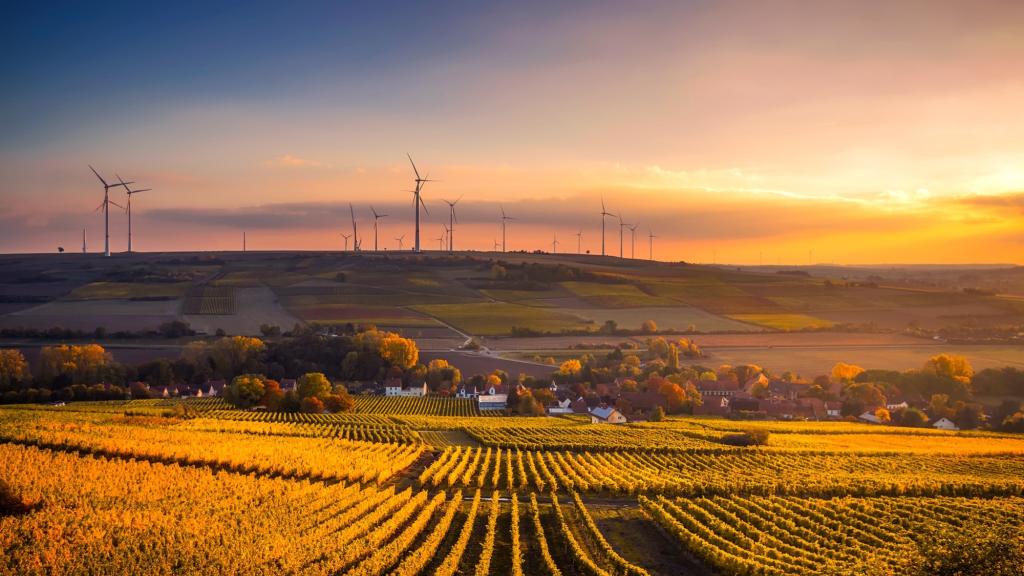The image captures a stunning landscape at sunset, bathed in a warm, golden glow. The sky, brilliantly colored with hues of orange and blue, is highlighted by long flat clouds, with the darkness beginning to creep into the left corner. In the background, a wind farm with several windmills is perched atop an elevated area, almost silhouetted against the vibrant sky. Below, a vast expanse of farmland stretches out, featuring rows of golden crops and multiple fields in varying shades of green. These fields are flanked by a tree line in rich autumn colors of green and orange, interspersed with small white houses, barns, and perhaps other buildings. The entire scene exudes a warm and inviting tone, encapsulating the serene beauty of the countryside at dusk.